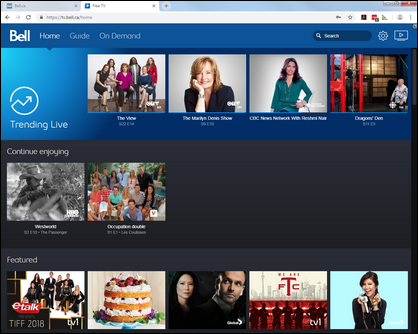This website advertisement appears to feature a service related to Bell Telephone, resembling streaming platforms like Hulu or Netflix. The predominantly blue website showcases white text for clarity and aesthetics. It is well-organized and visually appealing, with three rows of TV show thumbnails. Each thumbnail displays an image of the show and its characters or personalities, accompanied by brief descriptions underneath. The site features a "Trending Live" button for accessing popular content, along with several dropdown menus for seamless navigation. It also highlights shows you've recently watched, prompting you to continue viewing. At the bottom, there is a section for featured shows, ensuring easy access to notable content.